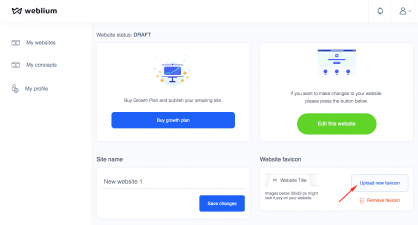The image is a screenshot of a web page with an all-white background. In the top left corner, the page is titled "Webulum." Below this title are three blurry sections: "My Websites," "My Concepts," and "My Profile." Towards the center-right of the image are two buttons side by side: a blue button on the left labeled "Easy Growth Plan" and a green button on the right labeled "Edit This Website." Centrally located at the bottom of the image is another blue button with the text "Save Changes." Additionally, a red arrow points to a rectangular button in the bottom right corner of the page, which reads "Upload a File."